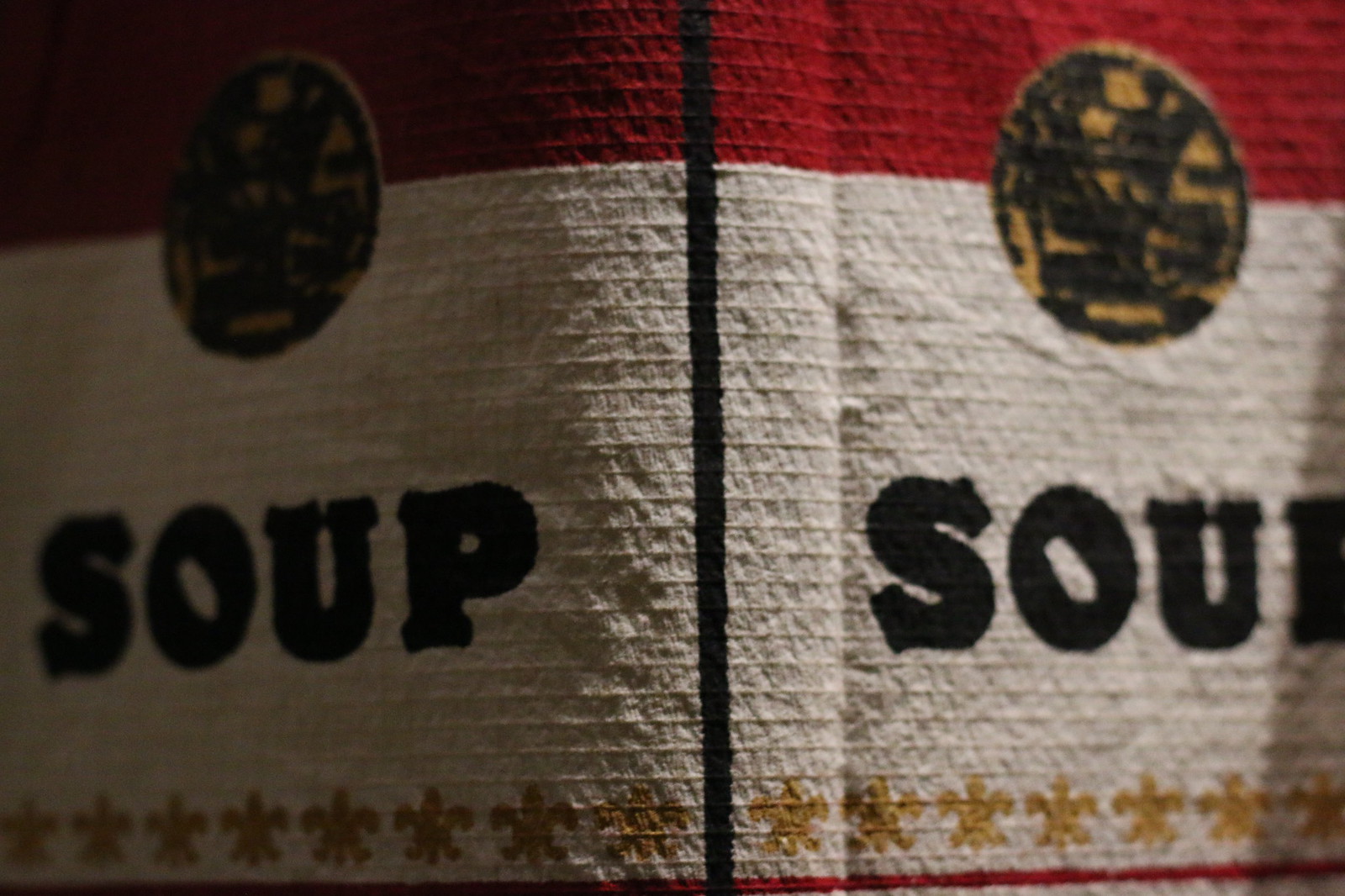This detailed image portrays an up-close photograph of an object designed to mimic the iconic Campbell's Soup can label. The object appears to be fabric fashioned into a book cover, positioned open to display both the front and back designs. The top portion of the fabric boasts a horizontal red band, reminiscent of the Campbell's Soup can, occupying approximately 10% down from the top. Midway through this red section, and extending into the white bottom half, lies a prominent gold and black round insignia. Each insignia features an orange-yellow background accented with several black splotches.

In the center of the white section, bold black block letters spell out "SOUP," with the right side showing the same but with the 'P' partially cut off. A distinct black line runs down the spine, separating the front and back covers. Along the bottom edge, a red trim frames both sides, complemented by a row of small gold stars or fleur-de-lis designs. Notably, the lighting highlights the front of the design clearly, while the back remains less illuminated, shrouded in partial shadow.